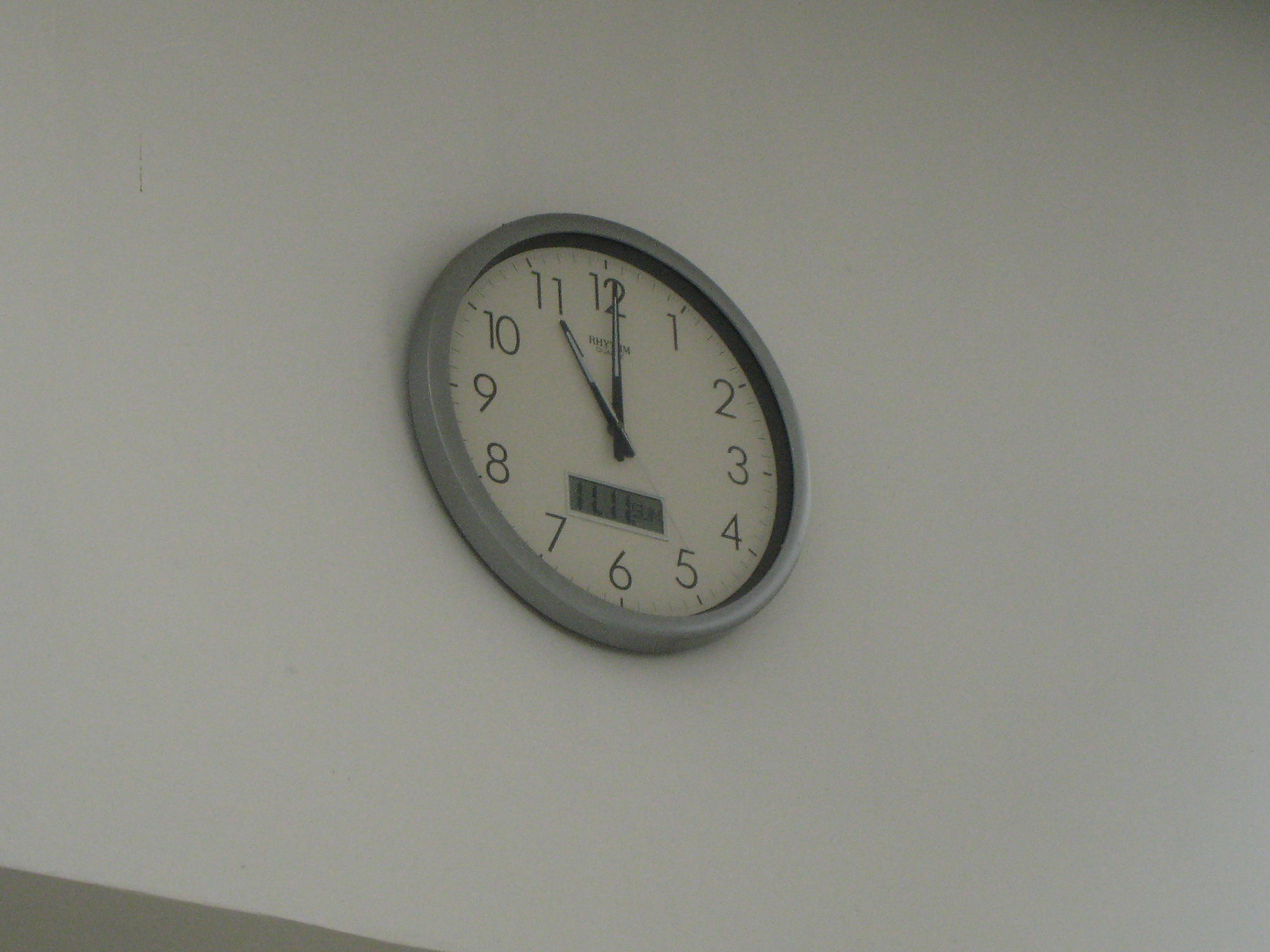This image features a round, schoolhouse-style clock mounted on an off-white wall. The clock's frame is gray, with a slight black border on the inside edge. Its face is white with black numbers and black hands, which have open centers at the tips, showing the time as 11 o'clock. Below the hands, there is a small rectangular digital screen displaying "11:11" in dark gray on a light gray background. This screen is located above the numbers 7, 6, and 5 on the clock face. The wall has a slightly darker, long triangular shape at the bottom left, contrasting subtly with the wall color.